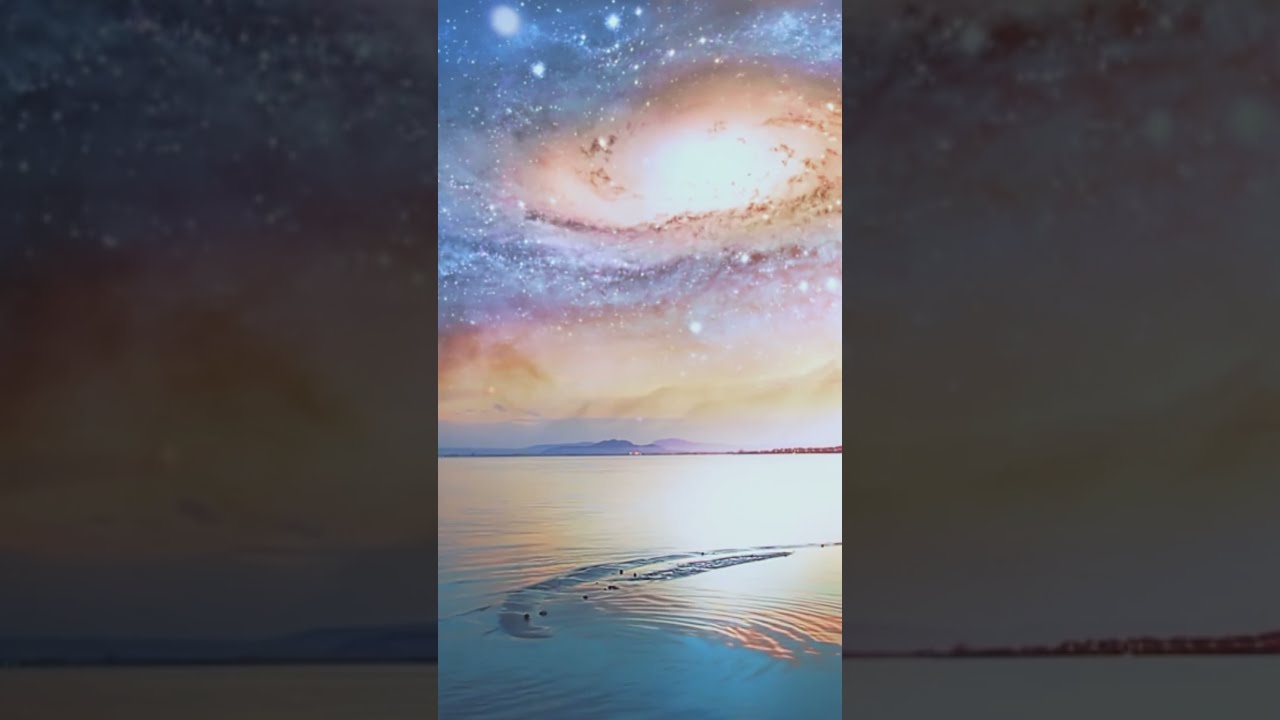The image is a highly detailed, photorealistic AI-generated artwork split horizontally into two distinct halves. The upper half features a breathtaking space scene with a spiral galaxy in the center, surrounded by vibrant blue and orange nebulae and a multitude of sparkling white stars. As the vibrant space scene transitions downward, it melds into wispy orange clouds near the horizon. Below this celestial display, the scene transforms into a terrestrial landscape with distant purple mountains and subtly rocky formations that could resemble a sandbar. The lower half of the image shows a purplish sky reflecting on a rippling body of water, possibly an ocean, which captures the nebulae’s vibrant colors. Additionally, there are orange swirls in the water and some indistinct floating objects. Flanking the sides of the image are opaque black borders, enhancing the focus on the central composition and providing a striking contrast to the vivid colors of the scene.